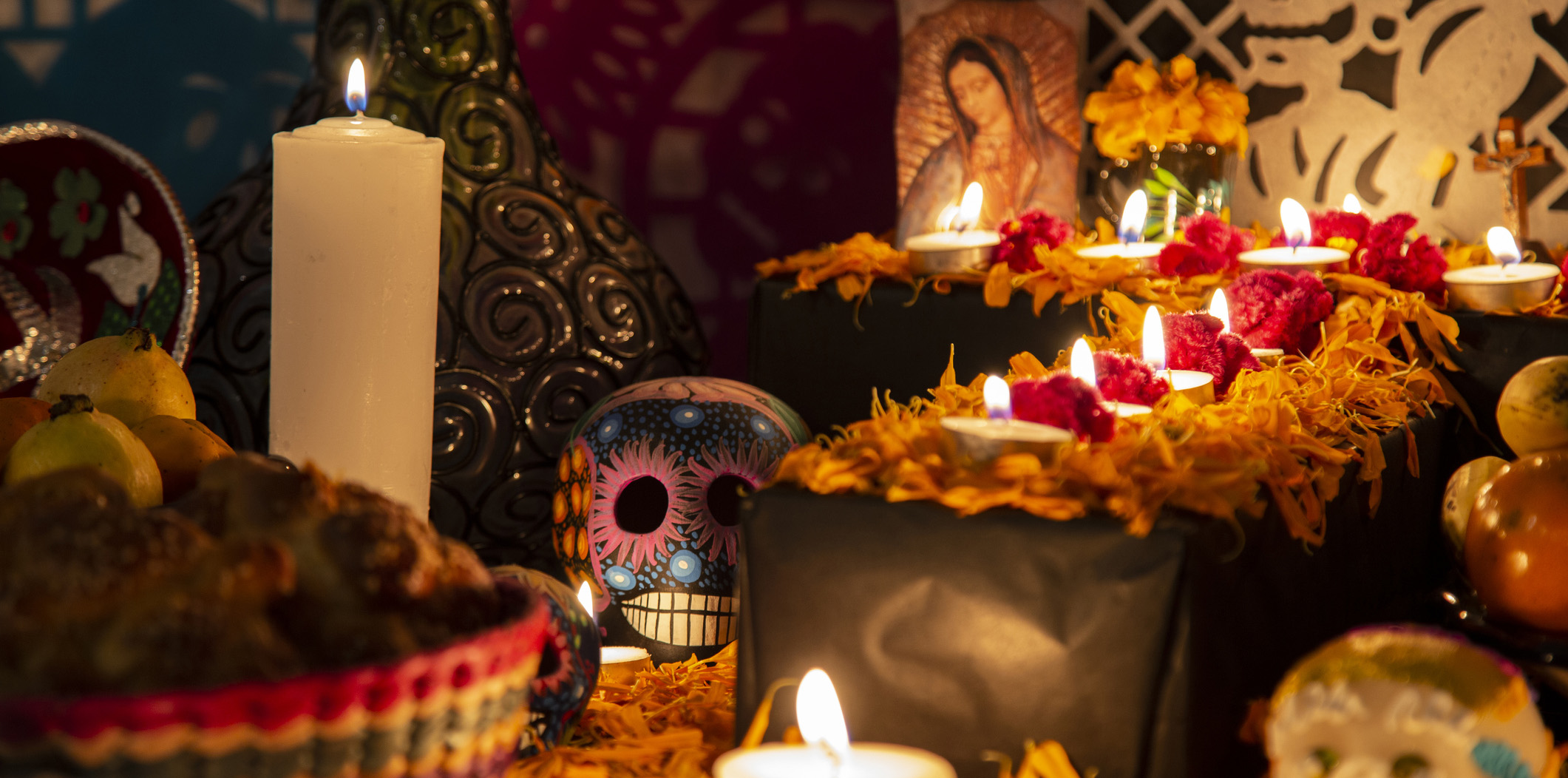This image depicts a richly adorned prayer station designed to resemble a chapel-like setting. The scene is dominated by a series of lit tea candles arranged against an orange and red floral backdrop, casting a warm glow over the dark surroundings. In the background, a picture of the Virgin Mary in a praying position is prominently displayed, adding a sacred aura to the space. To the right, a black and white design is partially visible, with a crucifix featuring Jesus situated in the upper right-hand corner. 

In the lower left section, a wicker basket rimmed with red, yellow, blue, and orange colors holds what appears to be potpourri. Behind this basket stands a large white wax candle with an ornate, scalloped metal design framing it. Centrally placed near this candle is a colorful, plaster-like skull adorned with vibrant patterns; its eyes are represented by black voids, its nose by blue bulbs, and its teeth by detailed black and white lines.

Yellow flowers and a black-and-white swirly glass item are scattered around, enhancing the mystical ambiance. The overall atmosphere is dark and eerie, with lighting provided predominantly by the glowing candles, giving the image a somewhat spooky, shrine-like appearance.